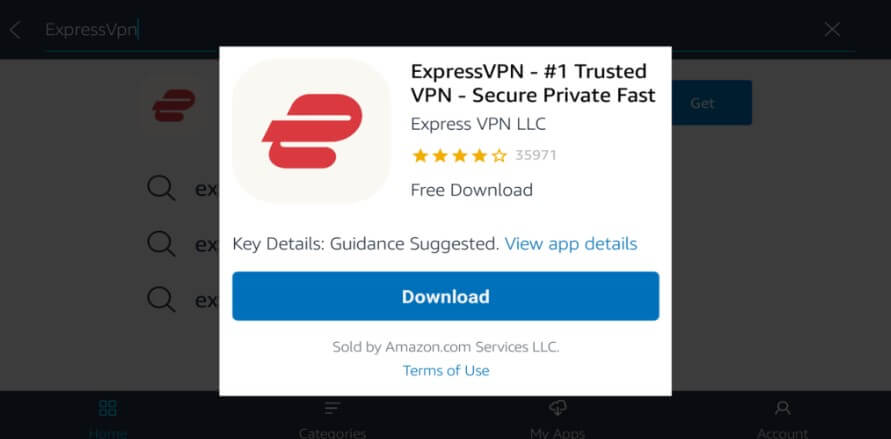The image shows a webpage with a gray overlay. On top of this is a white pop-up highlighting information about ExpressVPN. The pop-up features the company's name and slogan: "ExpressVPN: #1 Trusted VPN. Secure, Private, Fast." 

There is a logo on the left side resembling a stylized red letter "V" from "VPN". Next to the logo, text reads: "ExpressVPN LLC". Underneath, there's a star rating of 4 out of 5 stars, based on 35,971 reviews. 

Further down, a large blue button with white text offers a "Free Download". Other text indicates "Key Details" and "Guidance Suggested", with an option to "View App Details" in blue.

It is noted that the product is sold by "amazon.com services LLC" with "Terms of Use" linked in blue text. The predominant colors in the image are red, white, black, gray, yellow, and blue. The gray overlay lightly tints other underlying colors, giving a muted appearance to the whole webpage.